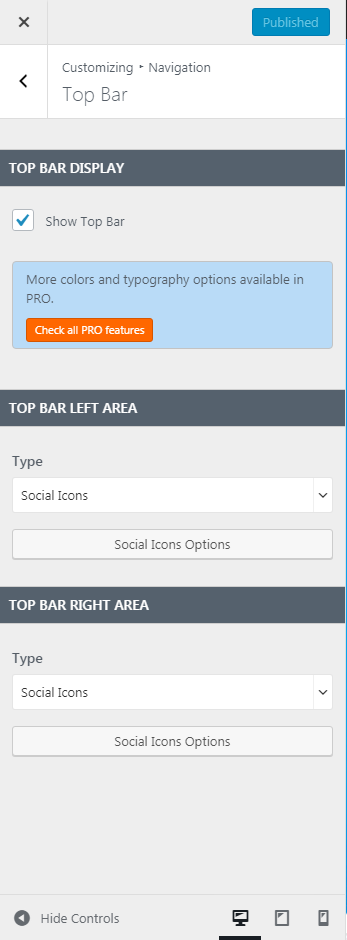The image depicts a user interface for customizing a website's top bar settings. At the top of the page, the heading reads "Customizing Navigation: Top Bar," indicating that the user is adjusting various aspects of the website's top bar. The background of the interface is a light gray, contributing to a clean and simple aesthetic. 

On the left side of the screen, a list of options is visible. The first option, "Top Bar Display," includes a checkbox labeled "Show Top Bar," which is currently checked. Below this option, there is a note mentioning that more colors and typography options are available in the pro version, highlighted by an orange button labeled "Check All Pro Features.”

Further down, the interface offers settings for "Top Bar Left Area" and "Top Bar Right Area." Both areas are presently set to display social icons, and users can choose which specific social icons to include. 

At the bottom left of the interface, there is a "Hide Controls" button, allowing users to simplify the view. On the top right, there's a prominent blue "Publish" button for saving changes. Additionally, a back button is available for users who want to navigate to different customization elements beyond the top bar. The overall design is simple and functional, with a square and rigid layout that prioritizes ease of use.